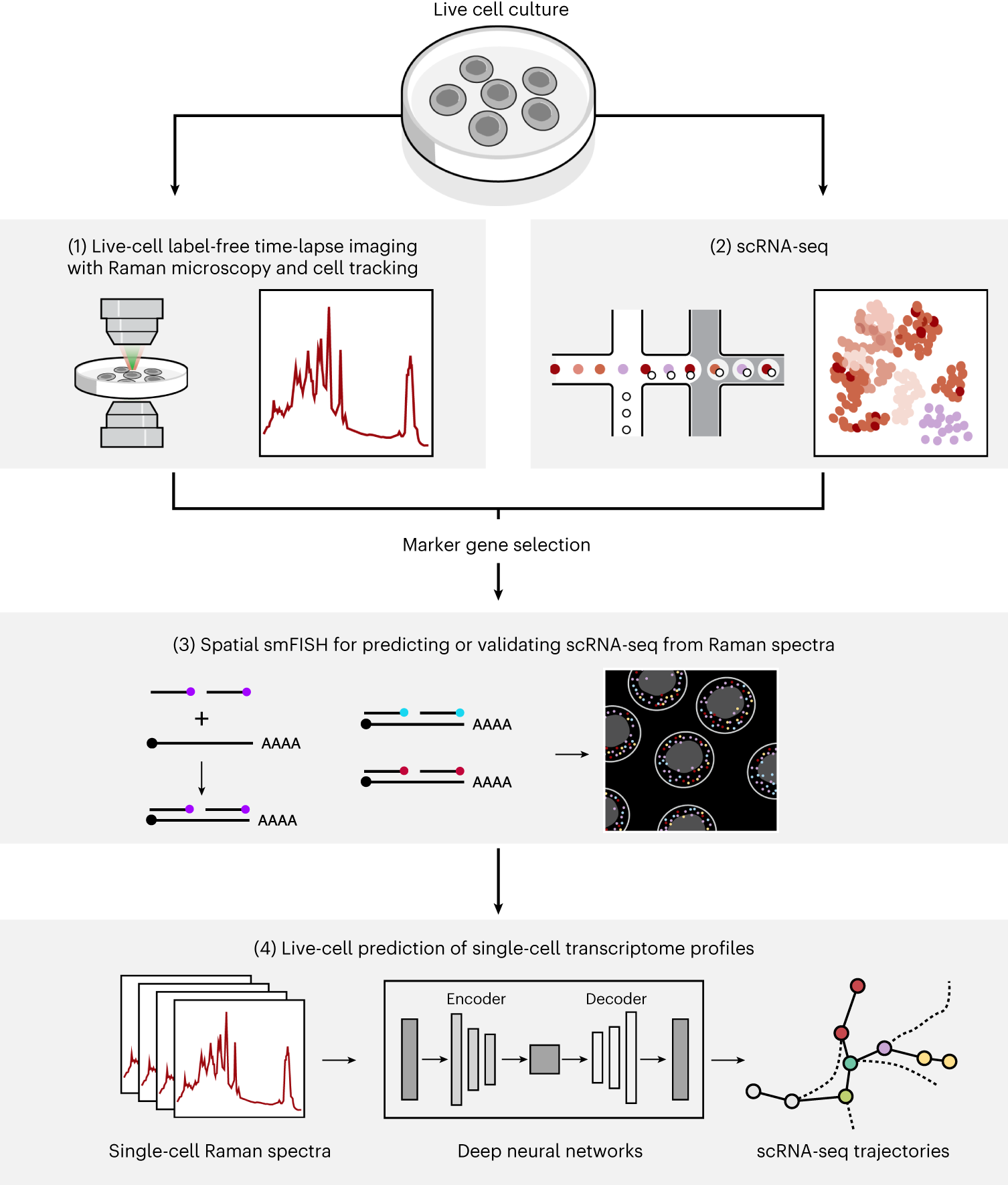The infographic provides a detailed representation of the processes and technologies used in live cell studies, divided into four sections. The top section depicts a petri dish labeled "Live Cell Culture," containing circular objects representing cells. Two arrows extend from the petri dish to subsequent sections. The left arrow points to a microscope lens image connected to a white box displaying a fluctuating red line, indicating 'Live Cell Label-Free Time-Lapse Imaging with Raman Microscopy and Cell Tracking.' The right arrow leads to an overview of cells with various colored dots, labeled 'SCRNA Sequencing.' Beneath this, another section titled 'Marker Gene Selection' is illustrated. The final part at the bottom shows boxes and bars indicating 'Live Cell Prediction of Single-Cell Transcriptome Profiles,' mentioning technologies like deep neural networks, single-cell Raman spectra, and SCRNA sequence trajectories. The infographic demonstrates the interconnected processes, from live cell cultures to complex predictive analytics, in cell studies.